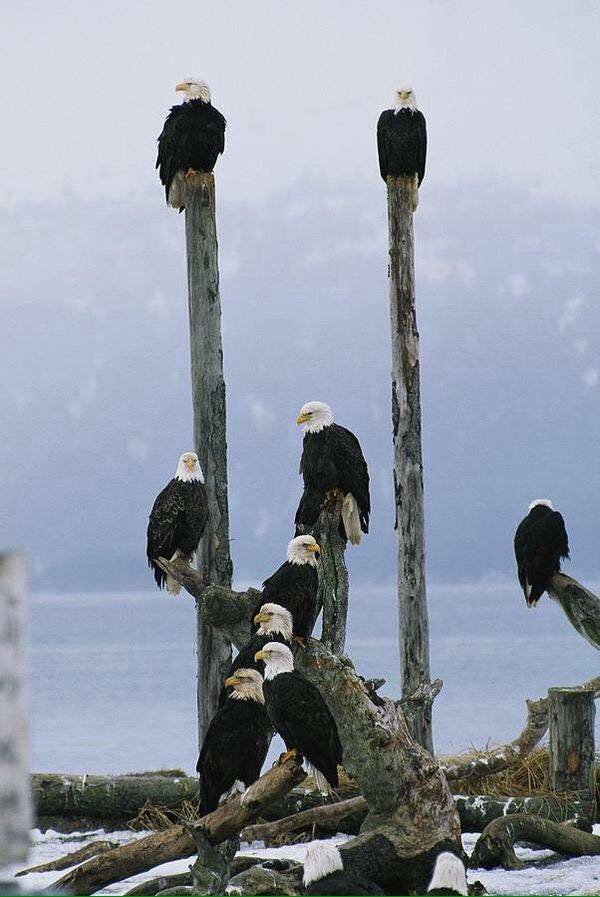This outdoor nature photograph features a stunning gathering of eleven bald eagles perched on various pieces of dead or dying wood near a body of water. The image is vertically oriented, about twice as tall as it is wide. Dominating the background is a slightly blurry, mountainous landscape, possibly snowcapped, beneath a clear blue sky. The middle ground of the photo reveals a serene lake, which transitions into a foreground covered in logs and snow, suggesting a chilly environment. 

Two prominent vertical logs stand nearly reaching the top of the photograph; each supports a bald eagle, identifiable by their white heads, black bodies, and yellow beaks. The eagle on the left log gazes leftward, while the one on the right faces the camera. Below and to the center, a more grounded and mangled piece of wood, resembling a tree root angled around ten o'clock, hosts the majority of the birds. Perched on this log are five additional eagles, contributing to the overall tally of eleven eagles throughout the scene. All eagles are perched, and none are seen on the ground. The logs and poles themselves are weathered and stripped, adding an aura of age and resilience to this beautifully rugged wilderness tableau.